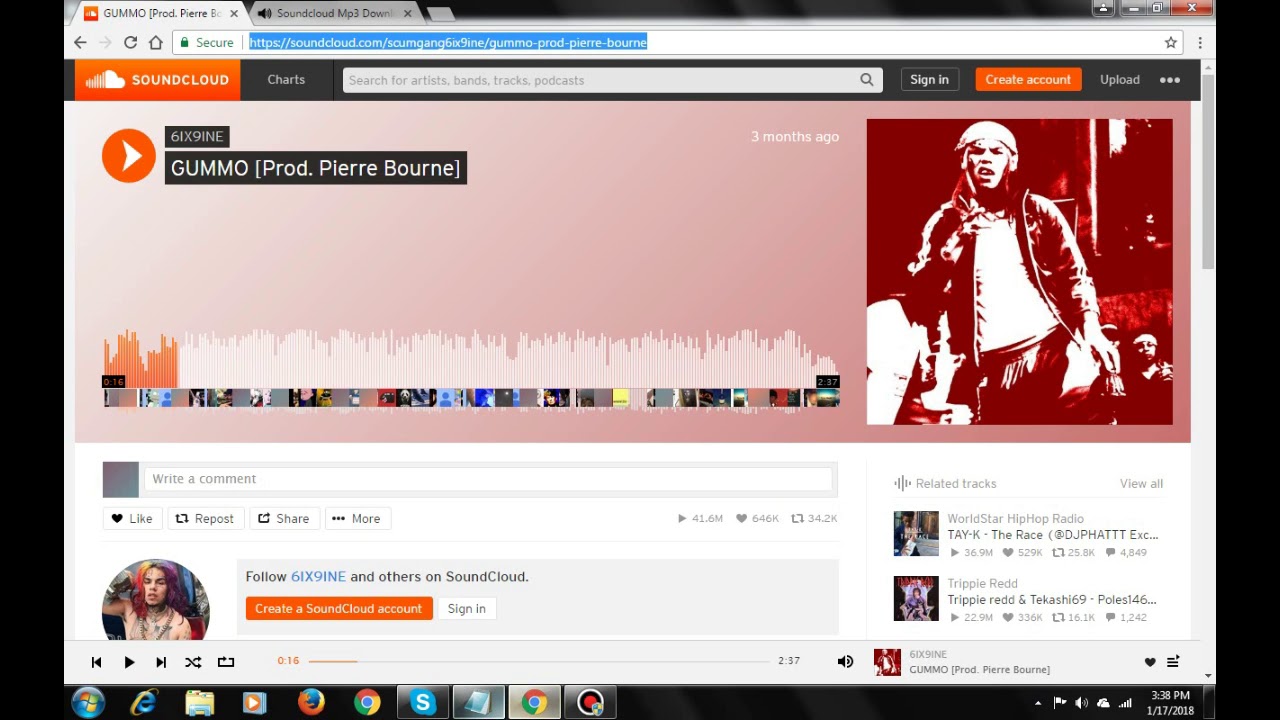In this detailed image, we can see a computer screen with a web browser open, displaying two tabs. Both tabs are associated with SoundCloud. The first tab features the iconic SoundCloud logo and is currently showcasing the artist 6ix9ine and his song "Gummo," produced by Pierre Bourne. Prominently displayed is the orange play button featuring a white arrow inside, indicating media playback functionality. 

The second tab is labeled "SoundCloud mp3 download," though the exact contents of this tab aren't visible. Observing the lower left corner of the screen, it's clear that this is a Windows operating system, identifiable by the presence of the Windows logo comprised of red, green, blue, and yellow colors. The taskbar also shows icons for Internet Explorer, a file folder, Windows Media Player, Firefox, Chrome, and Skype, indicating that Skype and Chrome are currently active. Additionally, a Notepad application appears to be open.

The SoundCloud page itself reveals related tracks, including WorldStarHipHop Radio and Tay-K's "The Race," which has an impressive 36.9 million plays. Another related track by Trippie Redd featuring Tekashi 6ix9ine has gained 22.9 million plays. The profile image for Tekashi 6ix9ine is also visible; he is depicted with his characteristic rainbow-colored hair, identifying him as a Mexican-American artist. Overall, the image captures an in-depth view of a SoundCloud page dedicated to Tekashi 6ix9ine's music, complete with related tracks and user interface elements.